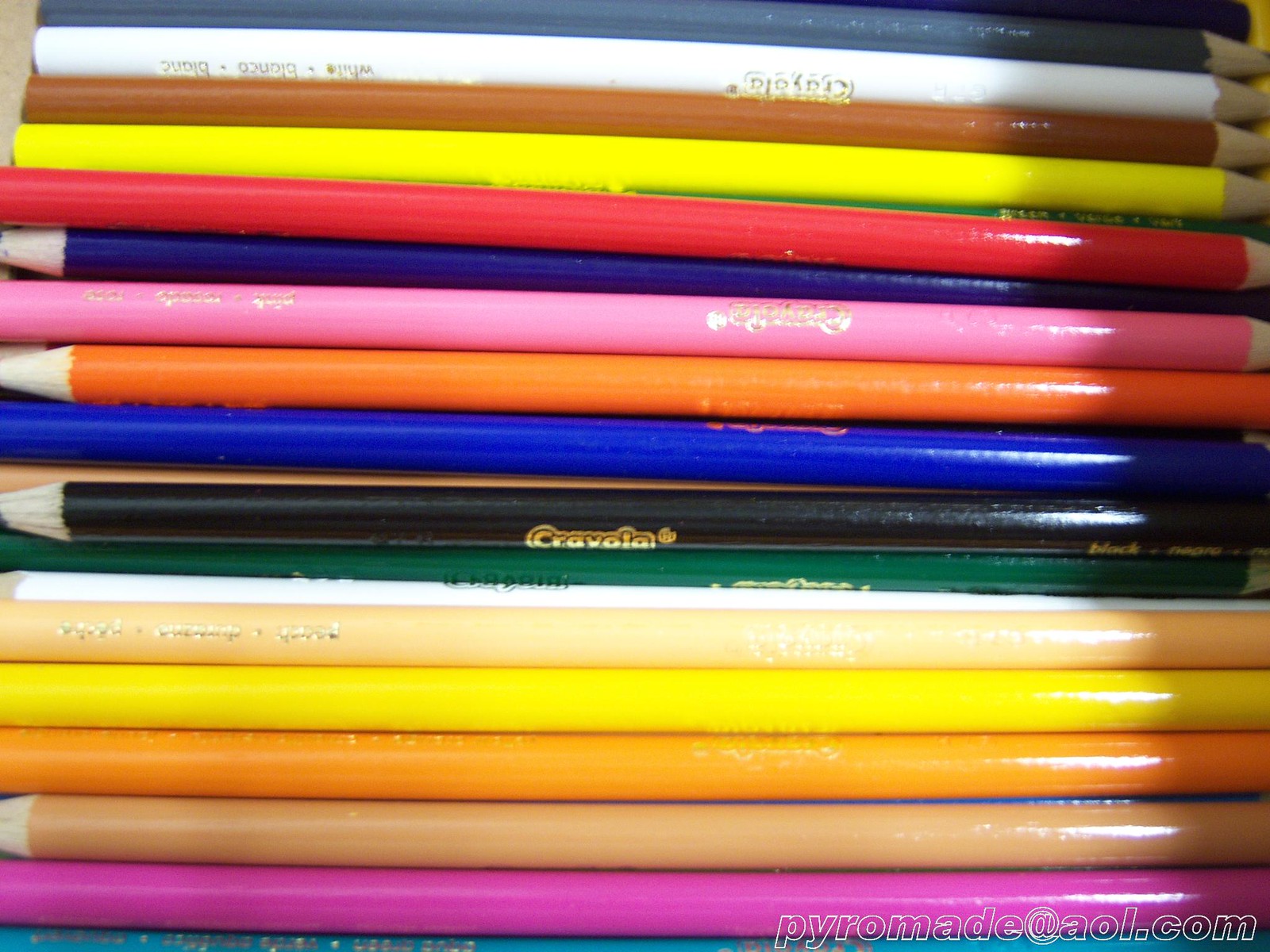This image displays a neatly stacked array of Crayola colored pencils nestled in a box, positioned horizontally with their tips hidden from view. The pencils, featuring a variety of vibrant colors such as white, brown, yellow, red, pink, orange, blue, black, green, purple, tan, and turquoise, form a strikingly colorful ensemble. The central, prominently placed black Crayola pencil is distinguished by its gold markings. The arrangement is illuminated with extra light casting a shadow toward the back, adding depth to the composition. In the bottom right corner, the text "PyroMade at AOL.com" appears in white bubble lettering, providing an identifiable signature to the image.